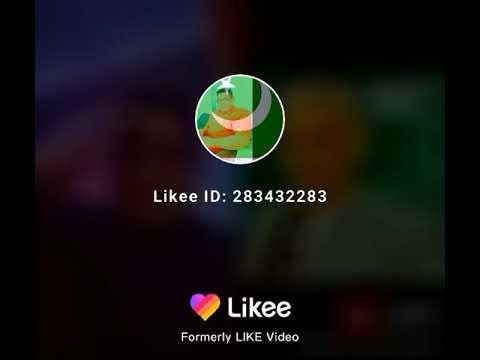The image is a detailed splash screen or about screen for a platform called Likee, spelled L-I-K-E-E. The layout is a nearly square rectangle with a complex visual design. The primary background is black, enhanced with a multi-colored filter that adds vibrancy to the overall look. 

At the top center, slightly above the middle, there is a white-outlined circle featuring an avatar. This avatar resembles a muscular man donned in a red tank top, flexing his bent arms. Superimposed over this man is a translucent white crescent moon, adding a unique thematic element to the image.

Directly beneath this circle, at the precise horizontal and vertical center of the display, the text "likee ID: 2834-32283" is prominently featured in white. This likely represents a specific user ID associated with the profile depicted in the avatar.

Finally, at the bottom center of the screen, a multi-colored heart icon, blending hues of purple, red, and yellow, is displayed. This icon is connected with the Likee platform and immediately below it, the name "Likee" appears in white text. Further emphasizing the platform's evolution, the text "formerly LIKE video" is placed below the Likee name, indicating a rebranding from its previous identity.